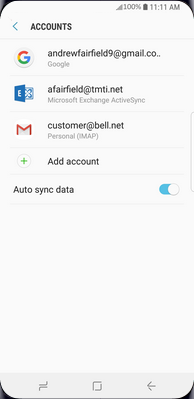**Screenshot of Android Interface with Email Account Details**

This image is a screenshot captured from an Android phone. The phone features distinctive design elements, with black ends and rounded corners that create a visually appealing, curved edge effect at the top left of the screen.

At the top of the screen, a status bar displays a full signal bar with "100%" indicated beside it, and a fully charged battery icon. The time is shown as "11 a.m.", separated by a thin line from the content below.

The main content begins with the Google icon followed by the email address "AndrewFairfield9@gmail.com" and the label "Google" underneath it. Below this, an icon resembling the letter "E" on a tilted square represents another email account. This account is listed as "AndrewFairfield@TMTI.net" under the label "Microsoft Exchange ActiveSync".

Further down, another section shows an email icon followed by "customer@Bell.net", labeled as "Personal (IMAP)". At the bottom of this section, there is an option to "Add account" and a toggle for "Auto-sync data" that is switched on.